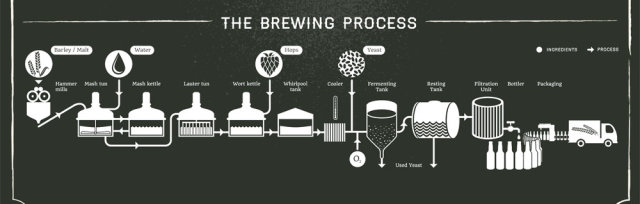The image presents a 2D computer-generated graphic with a dark green to black backdrop, explaining the brewing process in a clear, step-by-step manner. At the top, the text "The Brewing Process" is prominently displayed in white, flanked by two horizontal lines. Below this heading, a series of 2D-rendered illustrations, connected by arrows, outline the entire brewing cycle. The process starts with an illustration of barley or malt, moving sequentially through icons representing the addition of water, hops, and yeast. It then shows the fermentation in various tanks, followed by the distillation process. The final stages depict packaging, with bottles emerging from a circular tank, and conclude with a truck being loaded with the bottled products, ready for distribution. The clarity of the white pictorial elements and text against the dark background ensures that each phase of beer brewing from raw ingredients to shipping is clearly represented, making it an informative and visually accessible guide.